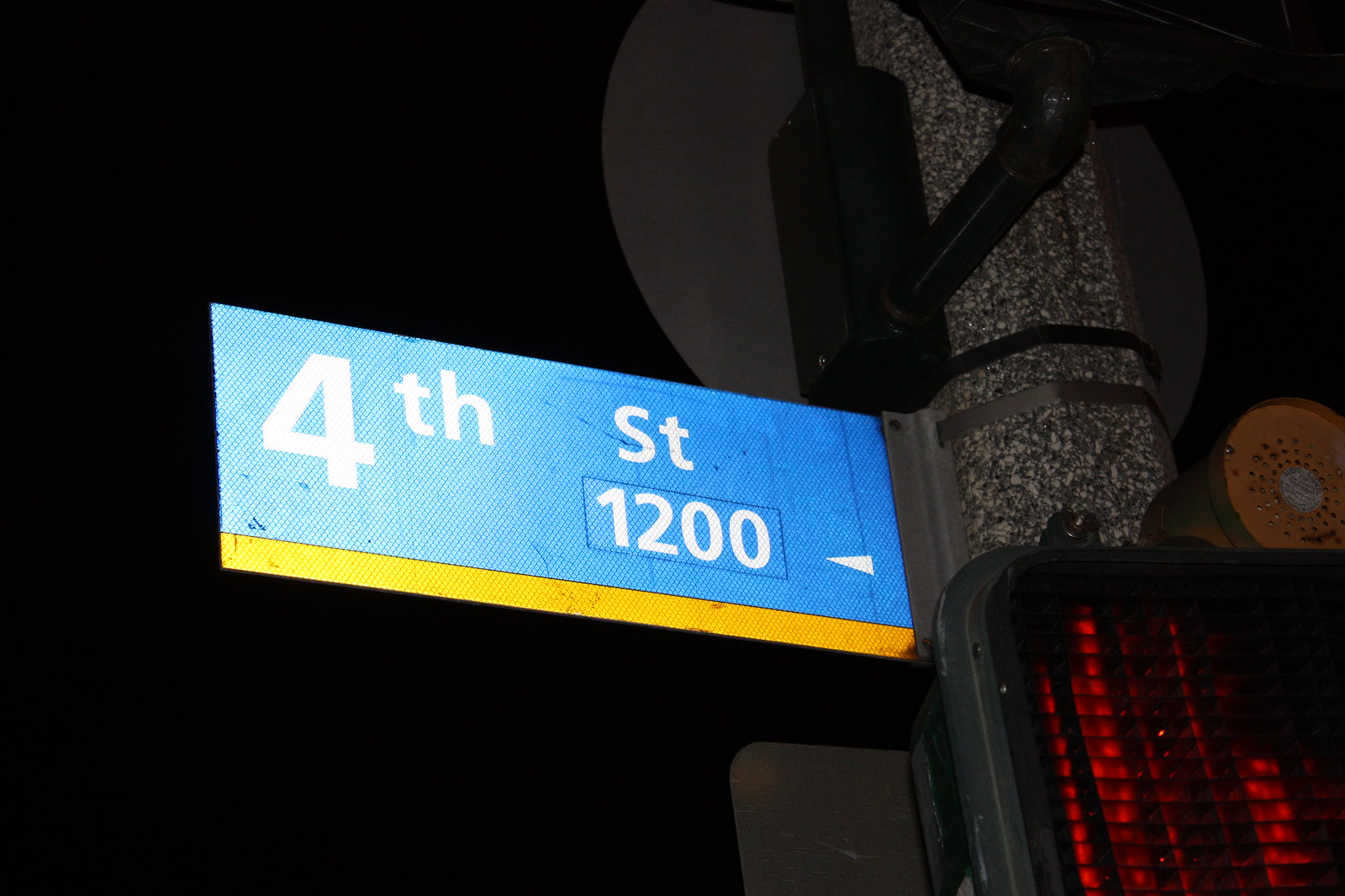This real-life photograph captures an urban street pole illuminated against a dark, nighttime background. The pole, prominently composed of a cement or granite-like material with specks of white, stands robustly. At its base, partially visible in the bottom-right corner, is a pedestrian button integrated with a crosswalk signal, currently displaying a red "stop" hand.

Ascending the pole, several elements adorn its surface. Notably, an orange, circular object resembling a speaker is affixed along with multiple metal bands. Attached midway, there’s the reverse side of a street sign.

The focal point of the image is a digital street sign extending from the pole. Displayed prominently in white text, it reads "Fourth Street." Below it, a blue rectangle with white text indicates "1200," accented with a small pointing triangle. Adjacent to this sign, an LED digital display features a blue background with a distinctive yellow bar at its base. 

Additional black equipment and various street signs decorate the pole, though they are less discernible. The stark contrast of the lit pole against the pitch-black backdrop accentuates the details and textures of the materials and elements present.